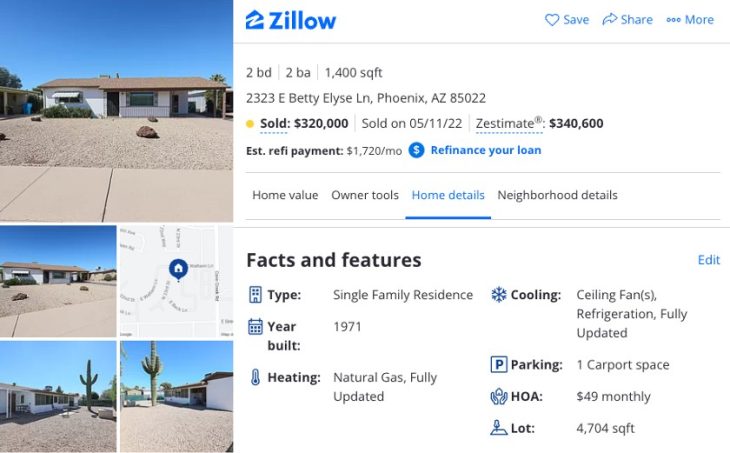This image is a screenshot from a Zillow listing page, formatted as a long rectangle with two distinct columns. The left column showcases images of the property, presenting a charming ranch-style house set against a vivid blue sky. The front yard is a quintessential desert landscape, predominantly covered in sand. You can also see a sidewalk running through the scene and a notable image of a cactus. One of the images features a map highlighting the property's location.

The right column contains the listing details. At the top, it prominently displays the Zillow logo along with options to save, share, or view more about the property. The listing describes a two-bedroom, two-bathroom home with 1,400 square feet of living space, located at 2323 East Betty Elyse Lane, Phoenix, Arizona, 85022. The home sold for $320,000 on May 11th, 2022.

Further details are organized under various tabs, with the "Home Details" tab currently highlighted in blue and underlined. Other tabs include "Home Value" and "Owner Tools." Under "Facts and Features," it specifies that the property is a single-family residence built in 1971, featuring natural gas, fully updated interiors, ceiling fans, and refrigerated air. It mentions that nothing about traditional air conditioning is found, emphasizing its location in a desert environment. The home includes one carport space and has a monthly Homeowners Association fee of $49. The entire lot spans 4,700 square feet.